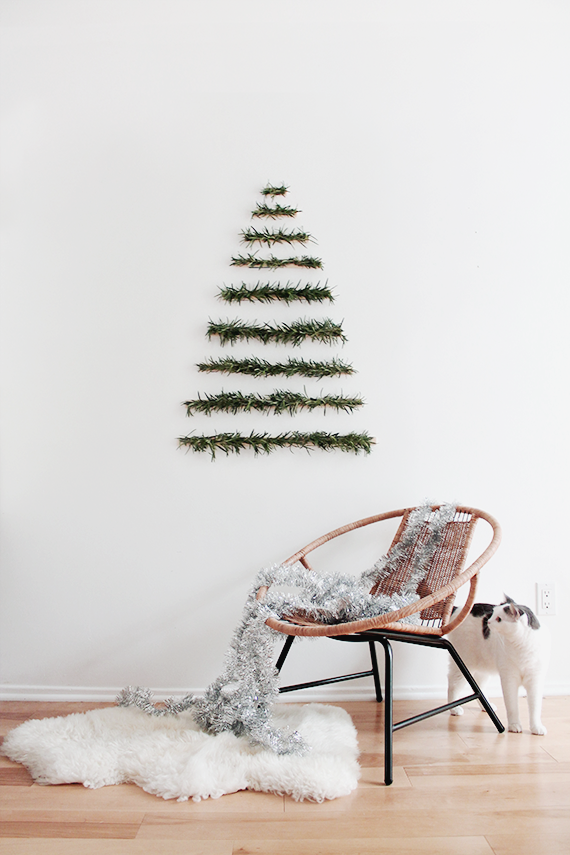The image depicts a tastefully decorated living room, featuring a Christmas-themed wall display and cozy furnishings. Adorning a clean, white wall is an arrangement of dark green strips of greenery, forming a triangular outline that mimics a Christmas tree. The rows of greenery gradually decrease in length as they ascend, creating a distinct tree-like shape with spaces between each strip. Below this festive wall decoration, the floor is a light brown wood, adding warmth to the scene.

In front of the wall stands a modern, round wicker chair with black steel legs, designed with a circular top resembling a hula hoop and a comfortable seat with a backrest. Draped over the chair is a string of shiny silver tinsel, cascading onto a thick, white sheepskin rug at the chair's base. Adding a touch of life to the setting, a black and white cat is positioned behind the chair, partly hidden but contributing to the cozy ambiance of the room.